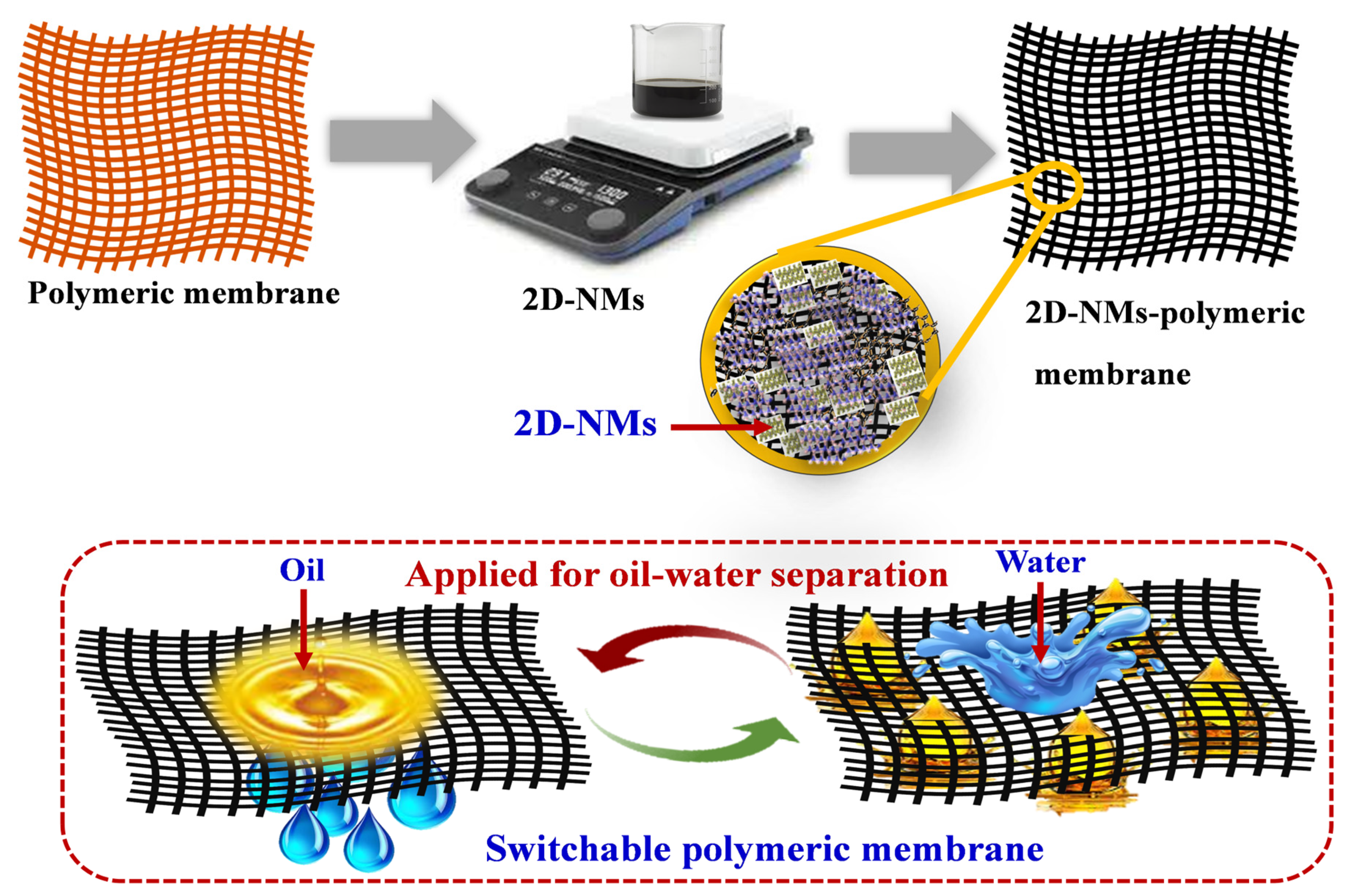The image is a detailed scientific diagram, likely intended for a textbook or a scientific journal, illustrating the function and application of switchable polymeric membranes for oil-water separation. The background of the diagram is entirely white, enhancing the clarity of the various components.

At the top, there are two polymeric membranes depicted. The left membrane is illustrated in red/orange color, with a gray arrow pointing to a digital style scale placed centrally, featuring a beaker with a black liquid. An arrow from the beaker points to the right membrane, colored black. Further to the right, there is an inset highlighted in yellow, enlarging a section of the black membrane to show a tightly meshed purple structure, labeled with descriptions such as 2D-NMs, emphasizing the membrane's microscopic details.

Beneath this, the bottom section features a large rectangular illustration outlined by a dashed red line. This section portrays two membranes from a horizontal perspective. The left membrane, associated with oil (indicated by yellow drips), shows the oil permeating it. The right membrane, associated with water (shown by a blue splash), demonstrates water permeation. Arrows in red and green form a circular pattern between the two membranes, underscoring the concept of fluid separation. Text annotations clarify that this system is a switchable polymeric membrane specifically applied for oil-water separation, illustrating the seamless exchange and selective permeability of the material for practical applications.